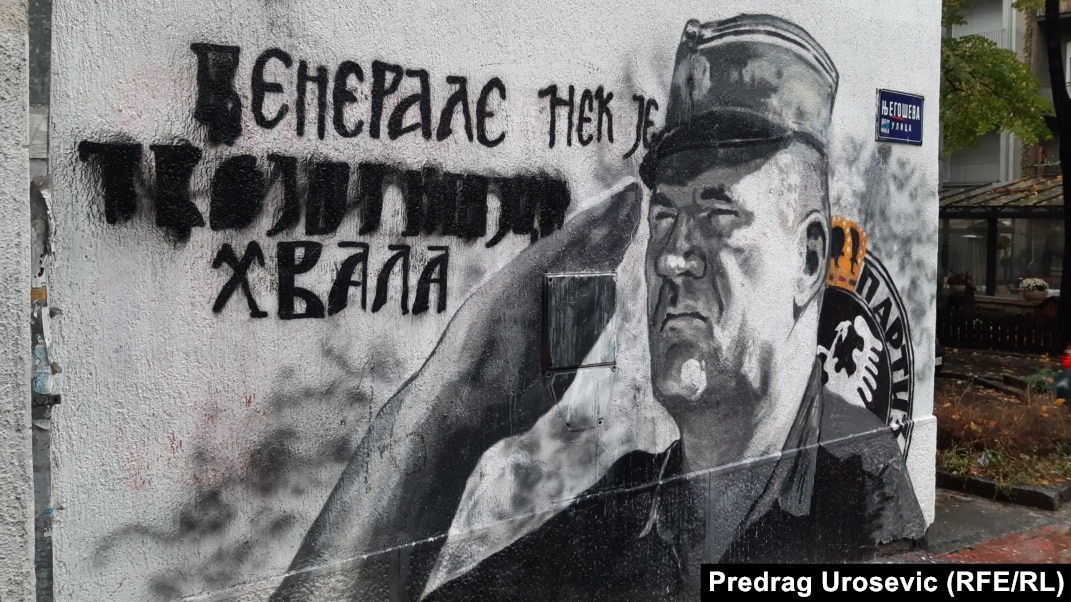This landscape photograph captures a detailed black-and-white outdoor mural painted on the side of a house. Dominating the scene on the top left is text in Cyrillic, indicating it is in Russian or another Eastern European language. In the center right of the mural stands a man in military garb, facing left with a serious expression. He is saluting and appears to be squinting, possibly due to sunlight. The mural—which seems to overlay a previous graffiti attempt—is intricately drawn and reflects a sense of concentration in the man's features. Below him, in the bottom right corner, is the text "Predrag Rusevich, RFE/RL." To the right side of the wall, near the edge of the mural, there is a handle or door lock beside a round object with partially obscured wording. In the background, a tree, leaves on the ground, and another structure with a small garden and window boxes can be seen, possibly indicating the mural's location resides near a restaurant.